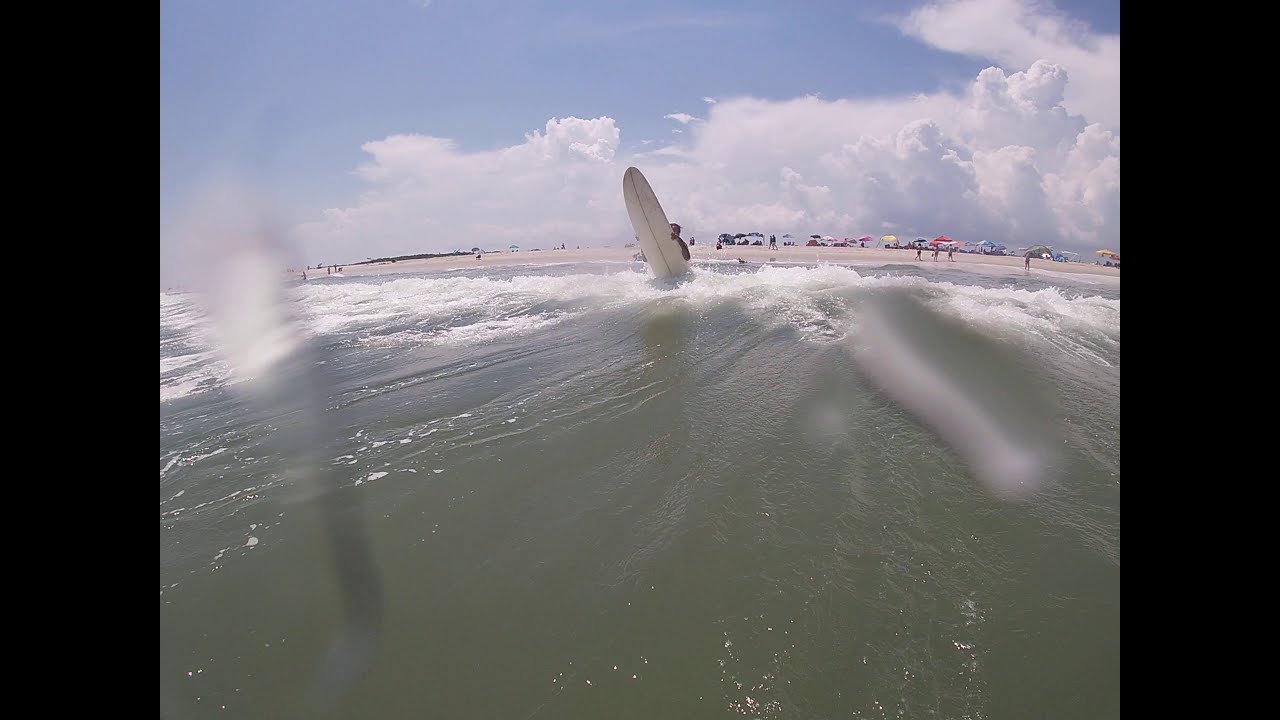This photograph captures a picturesque beach scene from the perspective of someone in the ocean, looking toward the shore. In the foreground, a man is wading into the water, holding a long white surfboard. The water, with a light green, glassy appearance, crashes into waves around his waist. It appears to be midday, with a predominantly cloudy sky stretching over the flat landscape, allowing an unobstructed view of the vibrant beach activity.

The beach in the background is lively, adorned with a myriad of colorful parasols and umbrellas in hues of pink, blue, red, yellow, and orange. The sand is dotted with numerous beachgoers leisurely walking about and enjoying their day, though the surfer is the sole individual depicted venturing into the ocean waters. Despite some blurriness and water drops on the camera lens, the center part of the image remains clear, highlighting the surfer and the dynamic, serene environment around him. The waves are gentle yet active, indicating a pleasant, sunny day ideal for surfing.